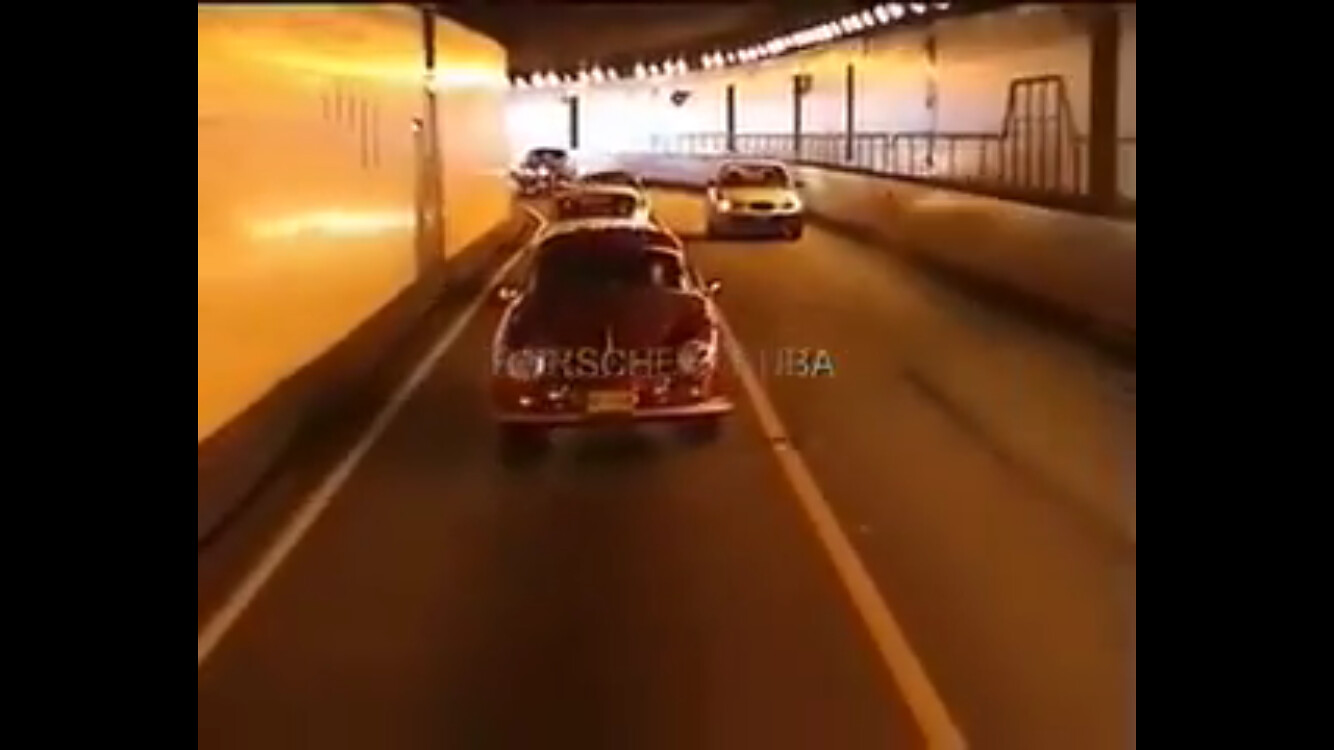This vintage photograph features a well-lit tunnel with a roadway running through it, bordered by wide black strips on either side. The tunnel's walls are light brown and adorned with numerous ceiling lights, providing ample illumination. On the right side, there's a half wall that transitions into a fencing structure, while a similar fence is visible in the background, adding an element of depth to the scene.

Prominently in the foreground is a red, classic car from a bygone era, leading a line of several other vehicles within the tunnel. In the opposite lane, a beige-colored car is visible, contributing to the nostalgic atmosphere of the image. The overall composition, with its combination of distinctive architectural elements and vintage automobiles, evokes a sense of traveling through time.